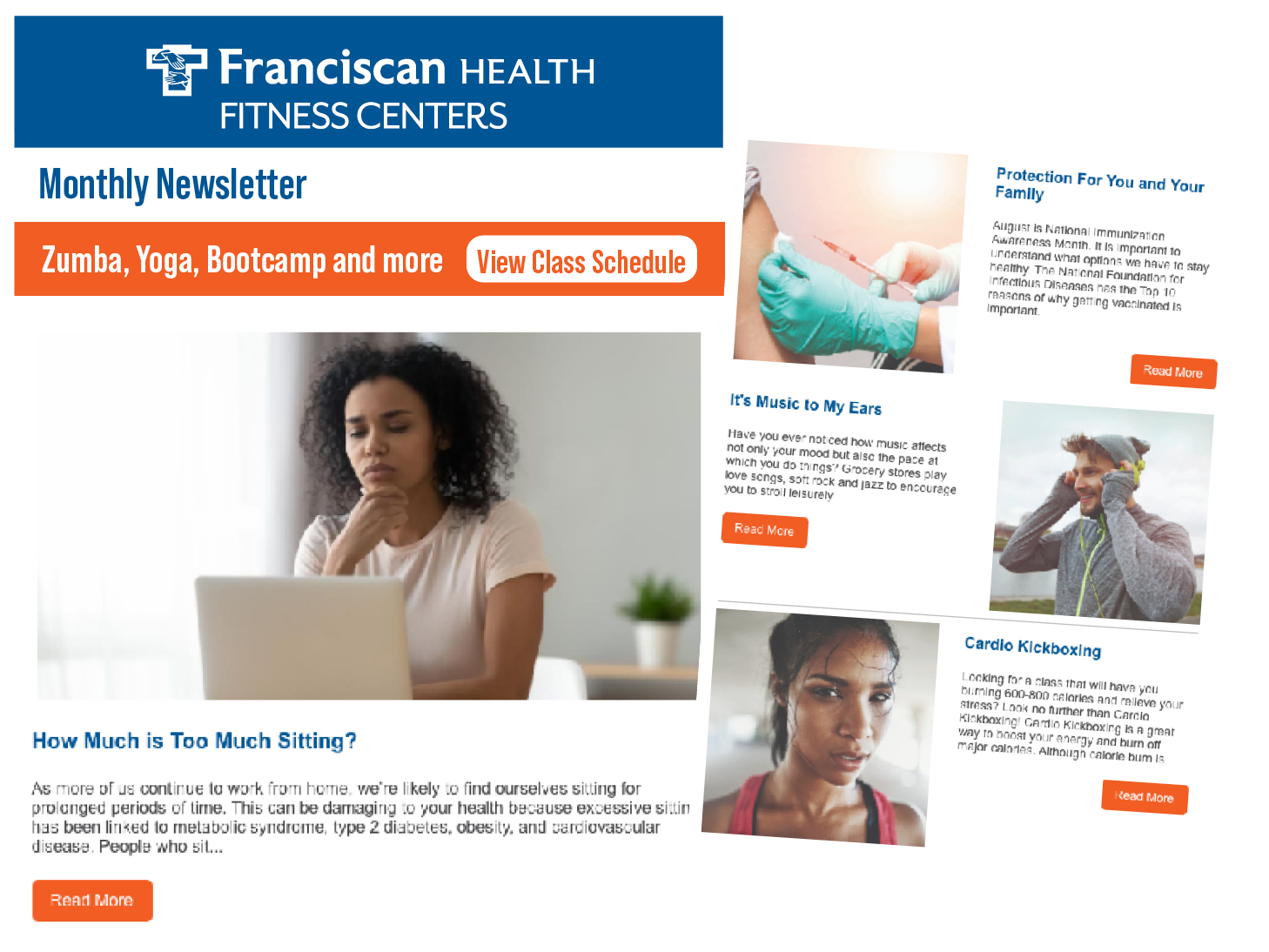This caption describes a detailed screenshot from the Franciscan Health Fitness Centers website. It’s split into two side-by-side pages with a plain white background, suggesting the screenshots were combined. The top section features a dark blue bar with the company name "Franciscan" in bold white text. The logo on the left includes a cross and two hands shaking or one helping the other, emphasizing a potential religious or community-oriented service.

Below this is the title "Monthly Newsletter" in blue text on a white background, followed by an orange bar that lists activities such as Zumba, yoga, and boot camp, with a "View Class Schedule" button beneath. An image of a woman resting her head on her hand while looking at a laptop introduces an article titled "How Much is Too Much Sitting?"

Adjacent to this, another blog post titled "Protection for You and Your Family: It's Music to the Ear," is also featured, with corresponding images for each article, enhancing the visual appeal and informative nature of the content.